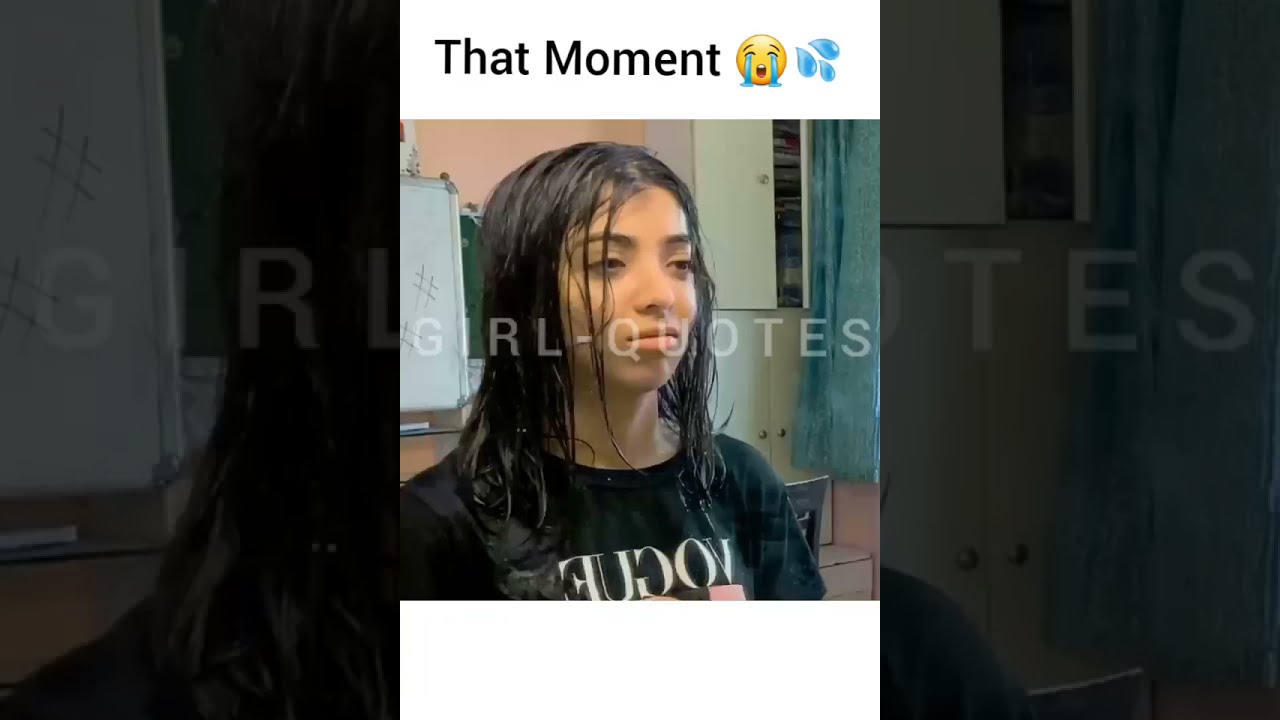This screenshot, taken from a smartphone, showcases a composite image where the central, full-color photo is bordered by grayed-out rectangles displaying the same image. At the top of the screenshot, a white bar with black text reads, “that moment,” followed by a crying face emoji and a water squirting emoji. Below this heading is an image of a young woman with wet, black hair, possibly of Mexican descent, wearing a black t-shirt emblazoned with the word "Vogue" in gold and white letters. The woman appears to be standing in a classroom, characterized by the whiteboard on her left and two cabinets on her right; the top cabinet is slightly ajar, revealing various books inside. Overlaid on the image, the transparent text “girl quotes” spans across her face. The overall scene, framed with a dark filter that contrasts with the brighter central photo, suggests a juxtaposition of emotions linked to the caption and emojis.